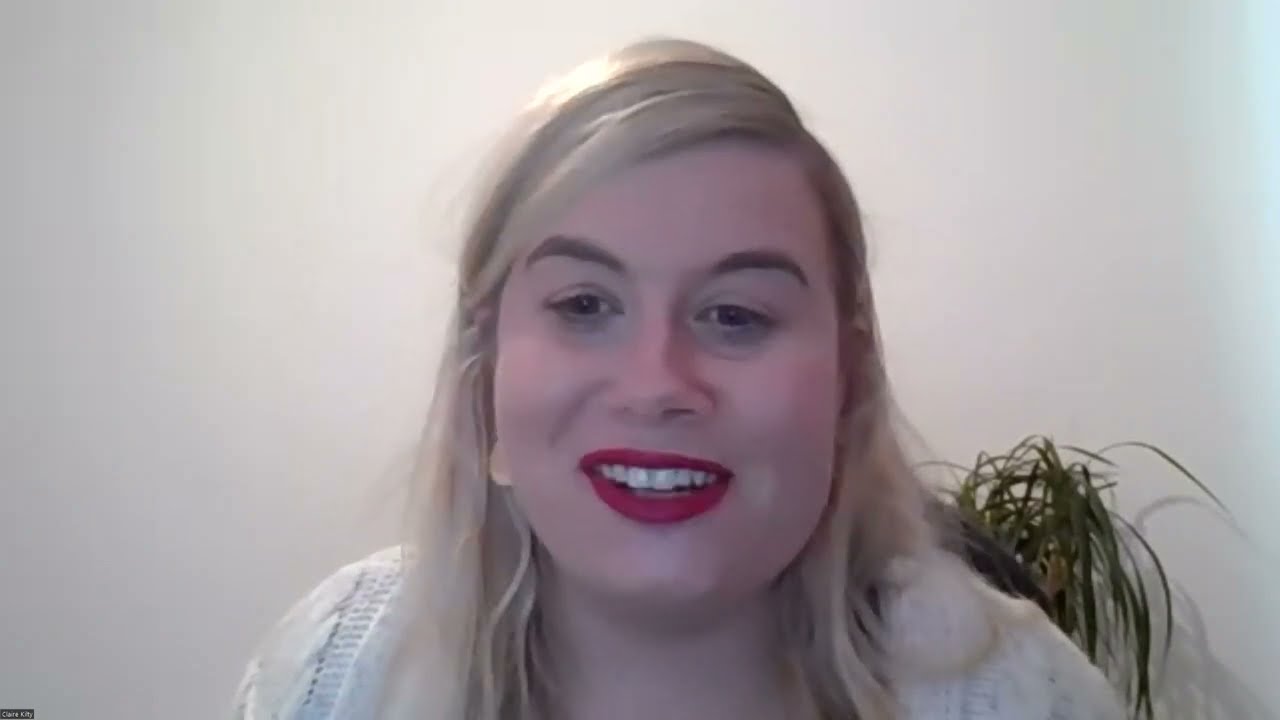The photograph depicts a young Caucasian woman in her mid to late 20s, seated centrally in front of a webcam, prepared for a video call or self-portrait. She has a fair complexion with a slightly pink tint and light blonde, shoulder-length hair, parted on her left side and swept over her forehead. Her hair extends just past her shoulders, catching a bit of light that creates a glare. She has dark arched eyebrows and dark eyes, which contrast with her bright red lipstick. The woman's round face is brightened by her open-mouth smile, revealing part of her top white teeth, giving the impression that she is speaking and smiling simultaneously. 

She is dressed in a white cable-knit cardigan, which she wears loosely over an unseen top. In the background, there's a plain white wall with a floor plant visible over her left shoulder. A faint rectangle with indistinct text or numbers can be seen at the bottom left of the frame, and the edge of a chair appears to her right.